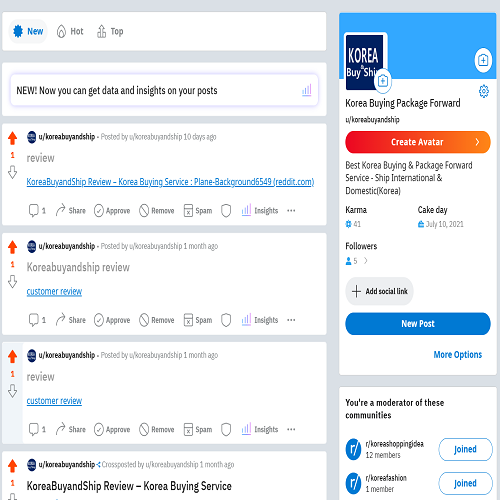A screenshot of a Reddit page under the "new", "hot", and "top" tabs at the top. Below, a notification banner reads, "new now you can get data and insights on your post". The main content displays several posts by the same user. 

The first post is titled "Korea Buying Ship Review" with a blue hyperlink below it that reads, "Korean buying service". The background information includes "playing background 6549" and the website "reddit.com". The same user has posted again with the title "Korea Buying Ship Review" and includes another blue hyperlink titled "Customer Review". 

Further down is another post simply titled "Review" with yet another link labeled "Customer Review".

In the upper-right corner of the page, there's a section labeled "Korea Buying Ship" with a logo followed by "Korea Buying Package Forward". Below this, there is an option to "Create Avatar". The description reads, "Best Korea Buying and Package Forward Service Ship International and Domestic". Additionally, there is a mention of "Korea cake day" on July 10th, 2021.